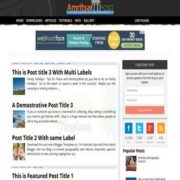The image features a composition with a black background and several elements dispersed throughout. At the top center, there is orange-ish text beginning with the letter "A," though the remaining characters are illegible due to the small size. Below the text, a blue line is present with some unreadable white text embedded within it, followed by a darker black font underneath.

The layout includes six clickable items, indicated in white, followed by an additional clickable item positioned further to the right. Adjacent to these elements is a purple advertisement featuring a mix of blue, white, and yellow hues.

Below the advertisement, there are three sections showcasing books, marked by black text. The titles, although partially readable, include: "This Post Title Three with Manual Labels," "A Demonstration Post or Tied Three," and "Post Title Two with Same Label." Another entry reads "This Featured [unreadable]." On the right-hand side, there are additional advertisements highlighted in black and pink colors.

Overall, while many of the details are too small and blurry to clearly discern, the image encompasses a mixture of text, clickable items, and colorful advertisements.